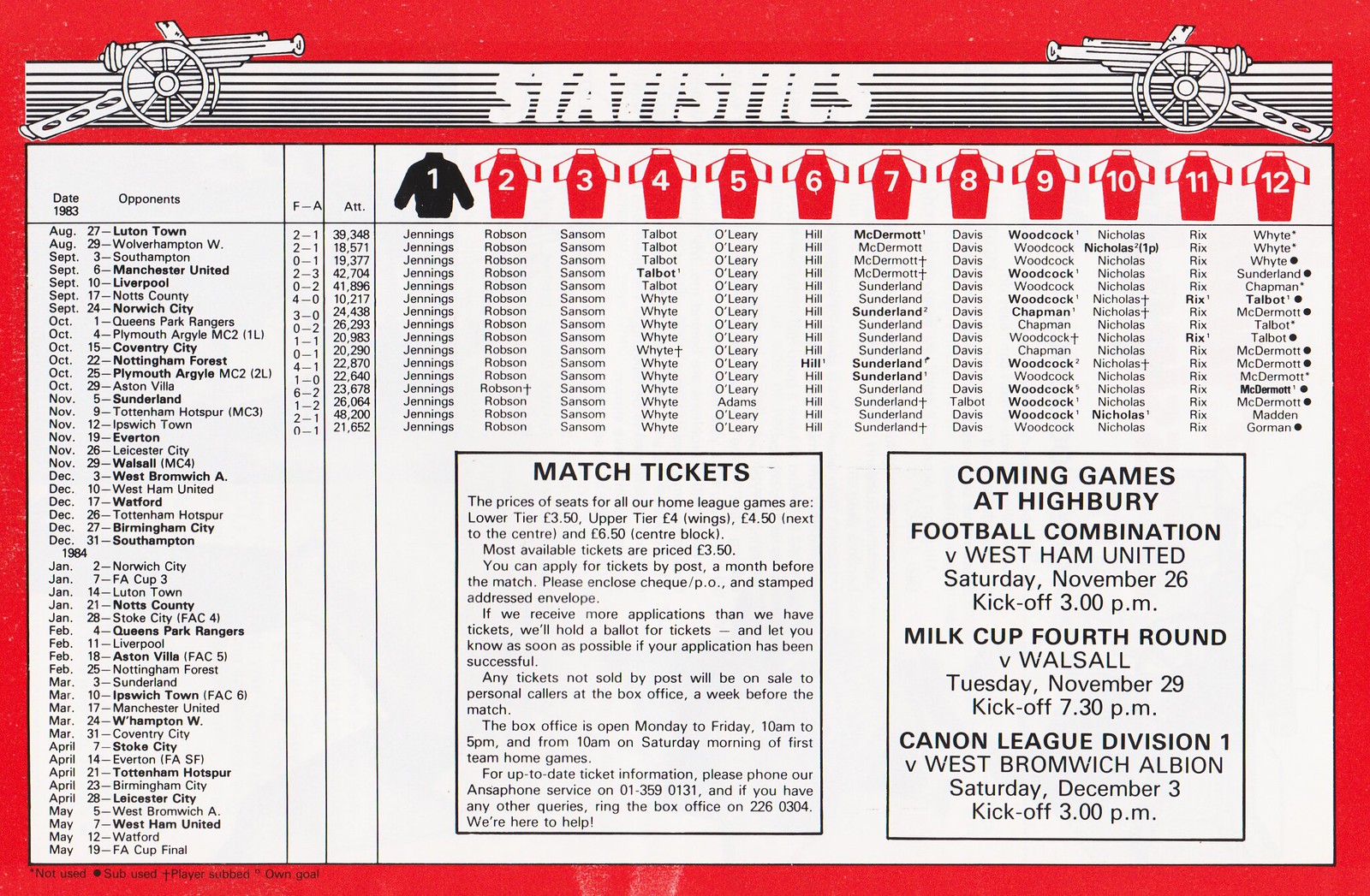The image is a scan of an old stat card or match ticket for a football club, featuring a historical style with a red border and a primarily white center with black text. At the top of the card, there's an illustration of two stylized artillery guns facing each other, framing the word "Statistics." The card displays information about player numbers, matches, and tickets. The jersey numbers 1 through 12 are depicted, where number 1 is black (likely the goalkeeper), and numbers 2 through 12 are red with white text.

Down the left side of the card, there are dates and opponents listed, while player names that correspond to their jersey numbers are aligned in columns across the card. Below this information, there are announcements for upcoming matches and ticket details.

The upcoming games mentioned are:
- Football Combination vs. West Ham United on Saturday, November 26th, with a 3 p.m. kickoff.
- MLK Cup 4th Round vs. Walsall on Tuesday, November 29th, with a 7:30 p.m. kickoff.
- Cannon League Division 1 vs. West Bromwich Albion on Saturday, December 3rd, with a 3 p.m. kickoff.

Ticket prices for home league games are segmented as follows:
- Lower tier: £3.50
- Upper tier: £4
- Wings: £4.50
- Next to the center: £6.50
- Center block: £6.50
Most available tickets are priced at £3.50. You can apply for tickets by post a month before the match, enclosing a check or postal order with a stamped addressed envelope. If ticket applications exceed availability, a ballot will be held. Unsold tickets will be available at the box office a week before the match, open Monday to Friday from 10 a.m. to 5 p.m., and from 10 a.m. on match-day Saturdays. For up-to-date ticket information, phone the ANSA service at 01359-0131 or contact the box office at 226-0304 for assistance.